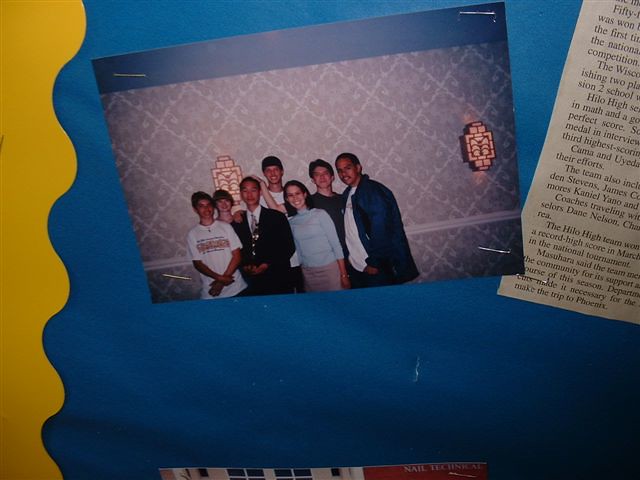The image depicts a detailed, colorful collage or bulletin board in an educational setting. Centered towards the upper middle, a color photograph shows a group of seven people, comprising both adults and children, standing side by side, looking directly at the camera. The people appear to be a mix of ethnicities, including an Asian man in a suit and a white woman, set against a hotel-like background with diamond-powdered lavender wallpaper and lights on the wall. The photo is mounted on a blue background with a scalloped yellow paper border to the left. To the right of the photograph, a partly visible newspaper clipping is stapled, featuring the words "high low high coaches high low high team" and "nail tech," though most text is cut off and unreadable. Below, another partially visible color photograph is also attached. The entire arrangement suggests a display meant for capturing memories and achievements.